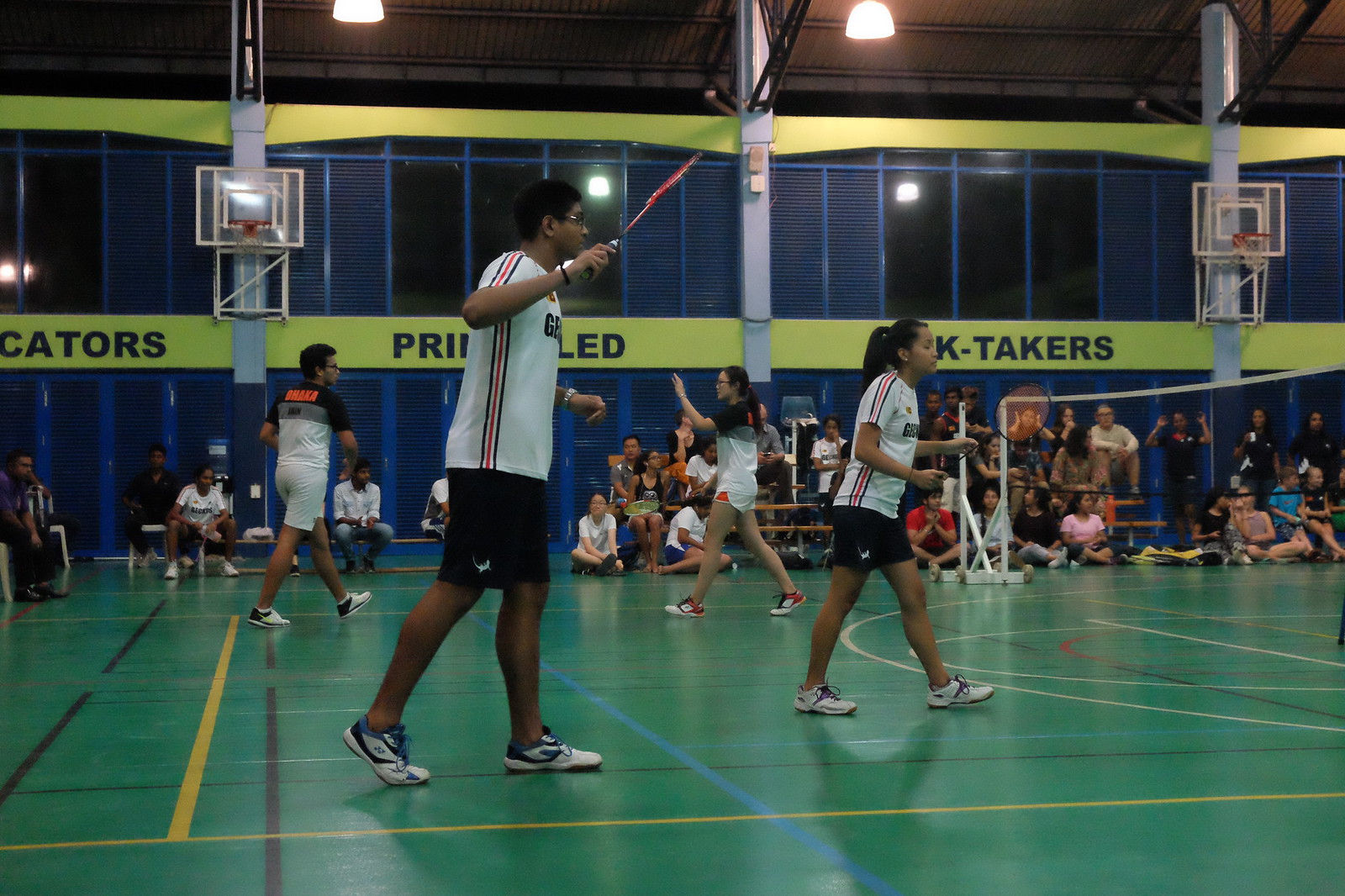This photograph captures an indoor badminton game set in a school gymnasium with a distinctive green floor. The image focuses on a foreground duo, a girl and a boy, who are significantly different in height. Both players are poised with their rackets; the girl holding hers lower while the boy raises his racket with his right hand. They are dressed in matching uniforms consisting of black shorts and white jerseys, denoting they are on the same team. Behind them is another team, distinguished by their different uniforms featuring white shorts and jerseys that are primarily white and gray with some orange detailing. The gymnasium is equipped with basketball nets, albeit folded up, and has a modest audience suggesting it is a small-scale event rather than a large auditorium setting. Spectators can be seen in the background, attentively watching the game.